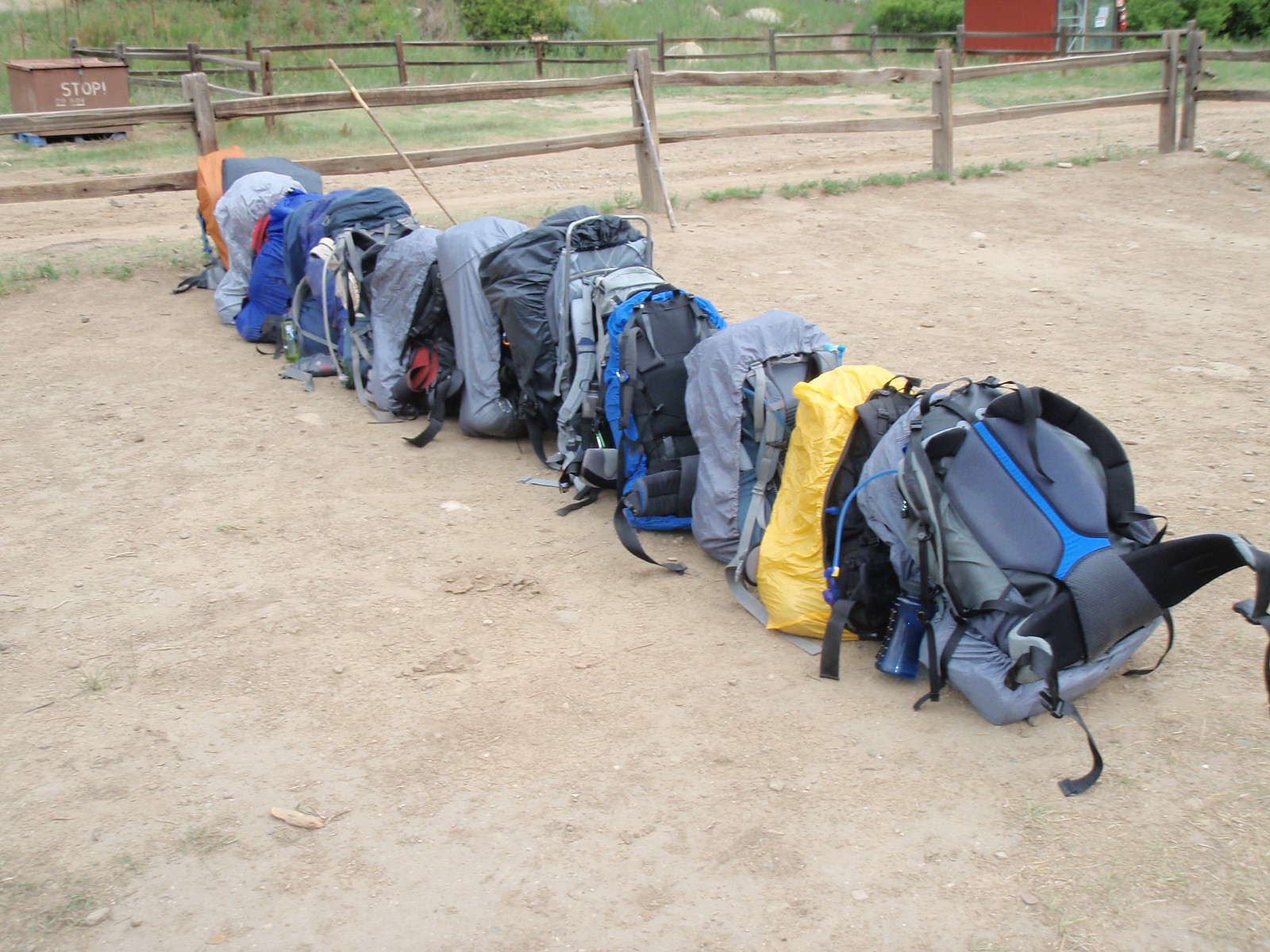This photograph, taken outdoors during daytime under a possibly overcast sky, showcases a dirt surface devoid of grass in the foreground. Lining this dirt ground are approximately a dozen assorted backpacks, predominantly in shades of gray and blue, with some distinct variations such as a yellow one and another with black and blue straps. These backpacks, seemingly designed for hiking with protective covers, are arranged in a row, some leaning slightly against a wooden fence composed of horizontal slats. Beyond this fenced area, a brown dumpster marked with the word "STOP" is positioned near another fenced section and a red outbuilding, resembling a large shed or small barn. The overall setting hints at a rustic, possibly rural environment, with additional details like a dirt road and sparse shrubbery contributing to the scene's ambiance.